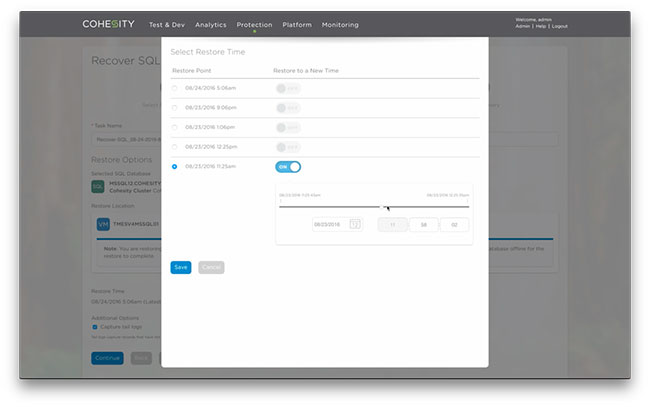This image is a low-resolution screenshot from a website, most likely viewed on a laptop, desktop, or tablet. The website features Cohesity, a company whose logo includes a green yin-yang styled 'S'. The navigation bar at the top of the page includes options such as "Test in Dev", "Analytics", "Protection", "Platform", and "Monitoring".

On the top right corner, although blurry, the text appears to include options such as "Admin", "Help", and "Logout", along with a possible user welcome message.

Highlighted in the image is the "Protection" section, displayed as a white pop-up window titled "Select Restore Time". The text inside the pop-up is difficult to read but seems to be "Restore Time" (misinterpreted as "Restore Pome" due to the blurriness). The list within the popup details several dates and times, prominently from August 24th, 2016, at various times like 5:06 AM and 9:06 PM, as well as subsequent dates like August 28th and 31st, and August 21st with corresponding times. Each date-time entry has an associated toggle option, though most are not activated. The exception is the last entry, which has an active toggle set for August 21st, 2016, at 12:23 PM.

To the side of these options, there is a slider bar designed to navigate through different dates and times for restore operations. Below the list of dates, there are action buttons, "Save" in blue and "Cancel" in gray.

Behind the pop-up window, partially obscured, is content that hints at additional features such as "Recover SQL”, “Restore Options", and "Restore Times", suggesting this interface is part of a software application focused on data protection and recovery settings. This screenshot likely represents a user interface element from a security or backup management software provided by Cohesity.